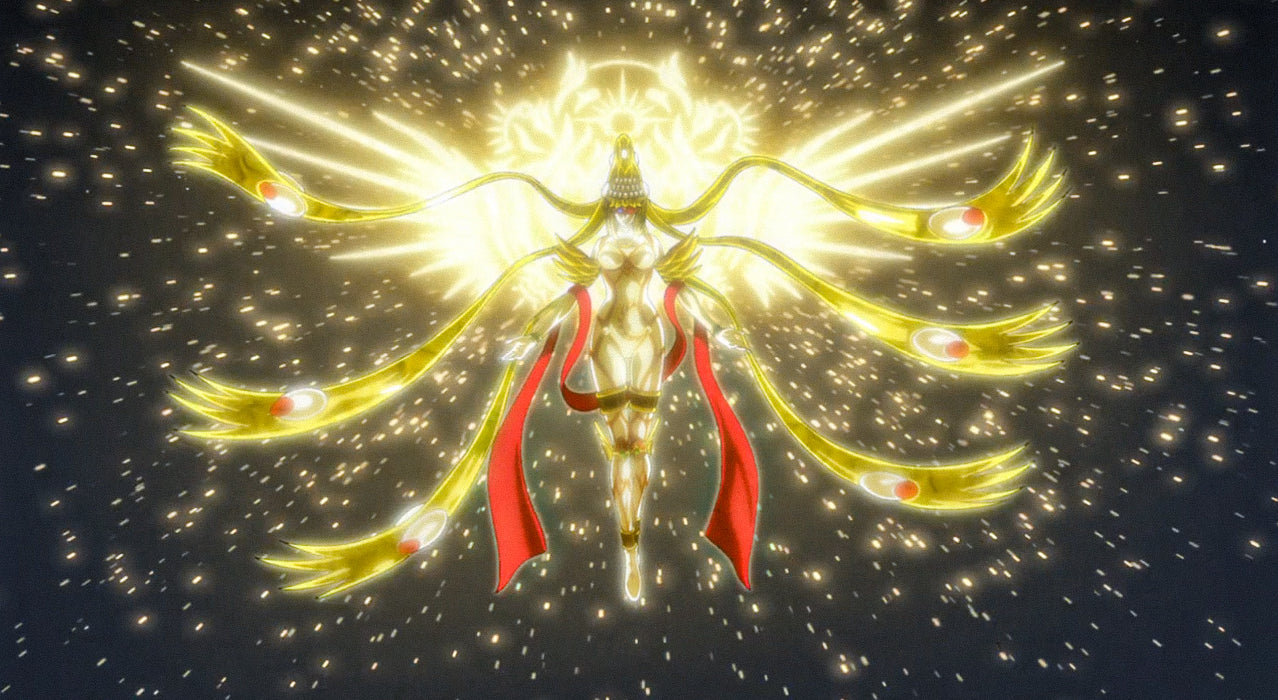The image depicts an intricate anime-style drawing with a black background, resembling a celestial or otherworldly scene. At the center is a majestic, curvaceous female figure, possibly representing a deity or goddess, adorned in white and gold attire. Her elaborate headdress, which emits a glowing golden light, features six long, ribbon-like extensions—three on each side—ending in white circles with red centers that resemble gemstones. These ribbons, appearing almost like flowing hair, cascade around her and intertwine with a red ribbon that wraps around her arms and legs, creating a dynamic, swirling effect. The figure's feathered, wing-like appendages extend from her upper arms, adding to her angelic or divine appearance. Surrounding her head are intricate designs forming halo-like shapes, with sparks of light radiating outward, creating a sense of motion and energy reminiscent of light speed through space. Behind her, a vivid emblem illuminates the scene, featuring ornate symbols that could be interpreted as a tiger, or perhaps an abstract representation of a deity like Vishnu. The overall composition, with its embellishments and ethereal lighting, gives the figure a powerful, almost mechanical presence amidst the star-streaked expanse.